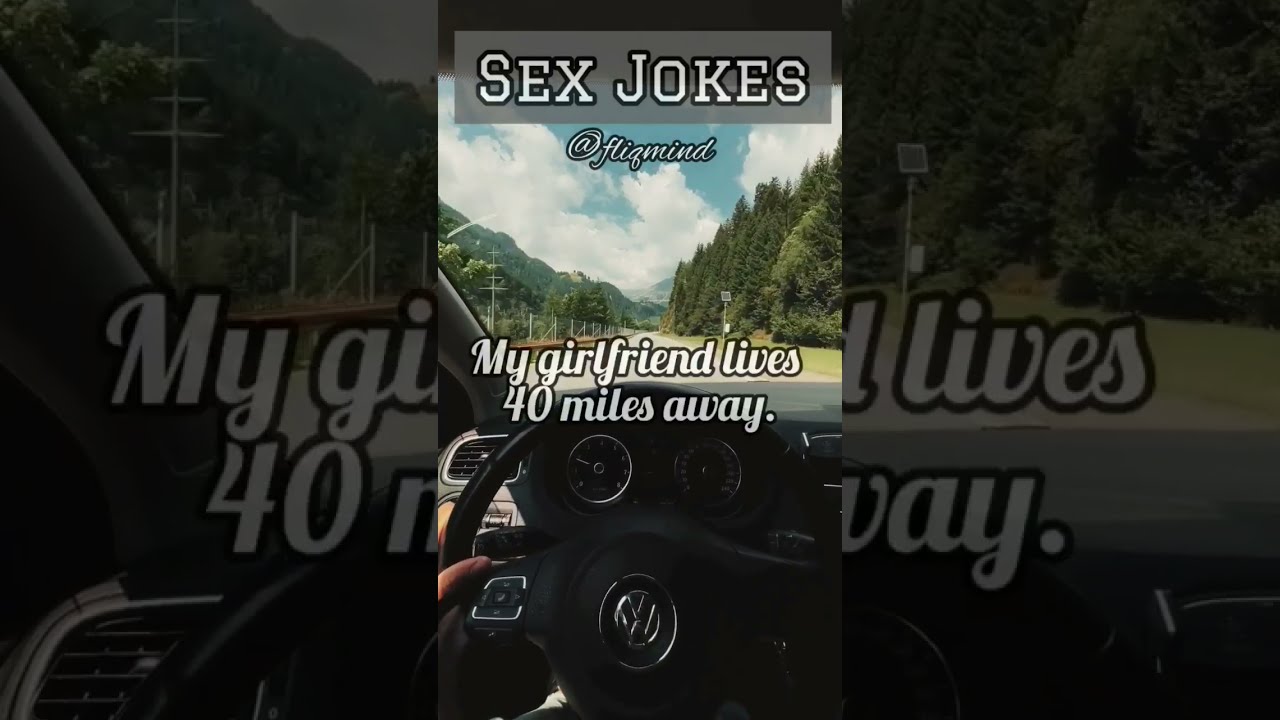This image captures a first-person perspective from the driver's seat of a Volkswagen, as evidenced by the logo centered on the black steering wheel. The scene is set on a clear, sunny day with a partially cloudy blue sky. Through the windshield, a winding road flanked by tall green trees stretches into the distance, suggesting a hilly or mountainous region. At the top of the screenshot, white capital letters in a gray border read "sex jokes," with the username "@fliqmind" written directly below it. In white cursive font, centrally positioned, the text "my girlfriend lives 40 miles away" adds a personal element to the image. The vehicle's dashboard reveals the speedometer, tachometer, and a glimpse of the driver's left hand on the wheel, indicating an active driving scene. The image is in portrait orientation, typical of a TikTok or Instagram reel.